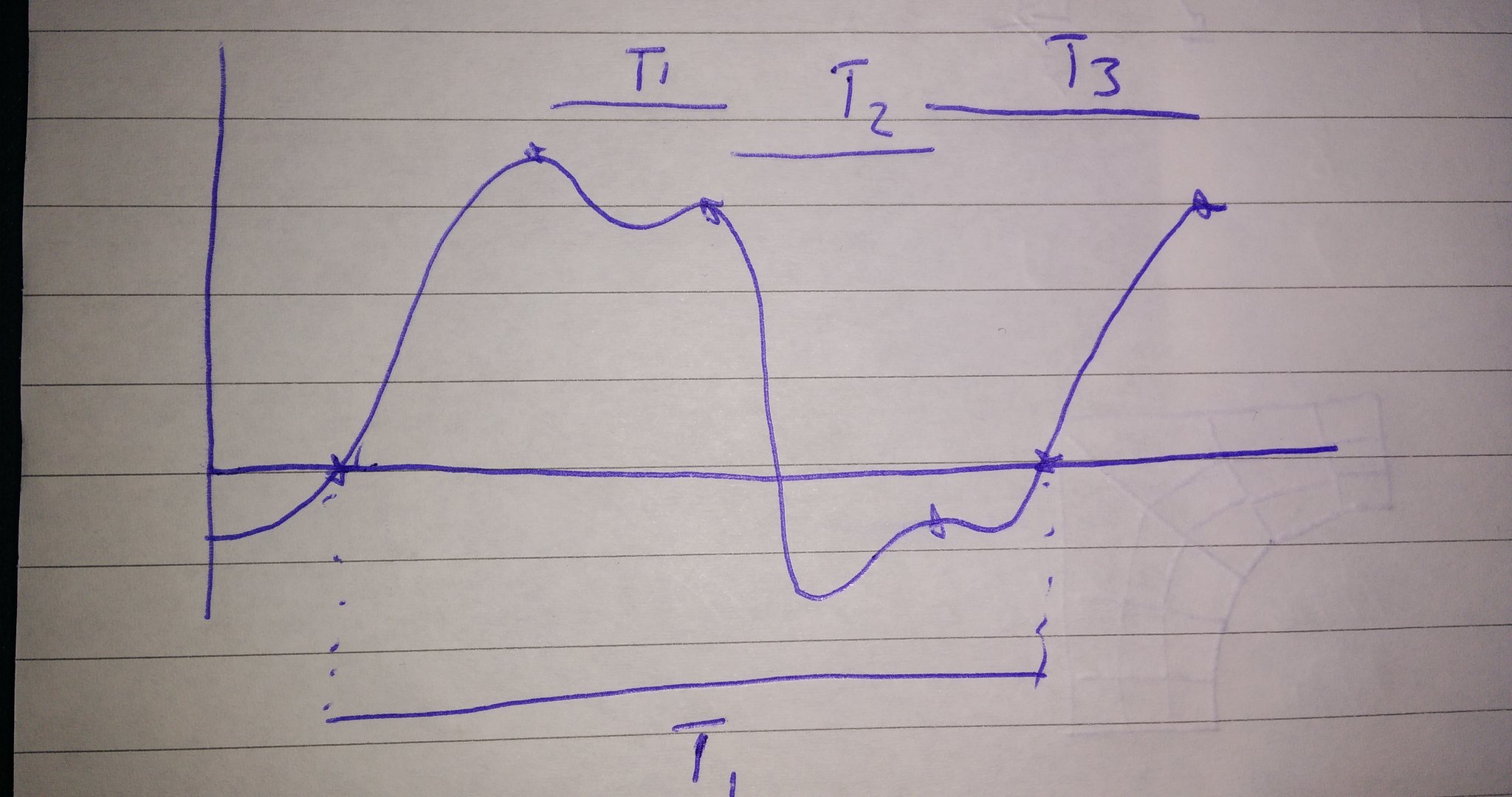This photograph showcases a piece of white notebook paper, identifiable by its classic blue horizontal lines designed to maintain straight writing and gauge writing precision, commonly used by school children. The sheet features writing in blue pen. At the very top of the page are three underlined titles: "T1" on the left, "T2" in the middle, and "T3" on the right. Below these titles, there is a graph depicting data points. The graph is structured with a horizontal line extending across the page, resembling a 'T' shape, with a vertical segment on the left side. The plotted data points create a curving line, consisting of six points that rise and fall in a wave-like pattern. Beneath the graph, directly under two of the base points, there are seven additional dots leading to another horizontal line extending across the page. The bottom-most annotation features the label "T1."